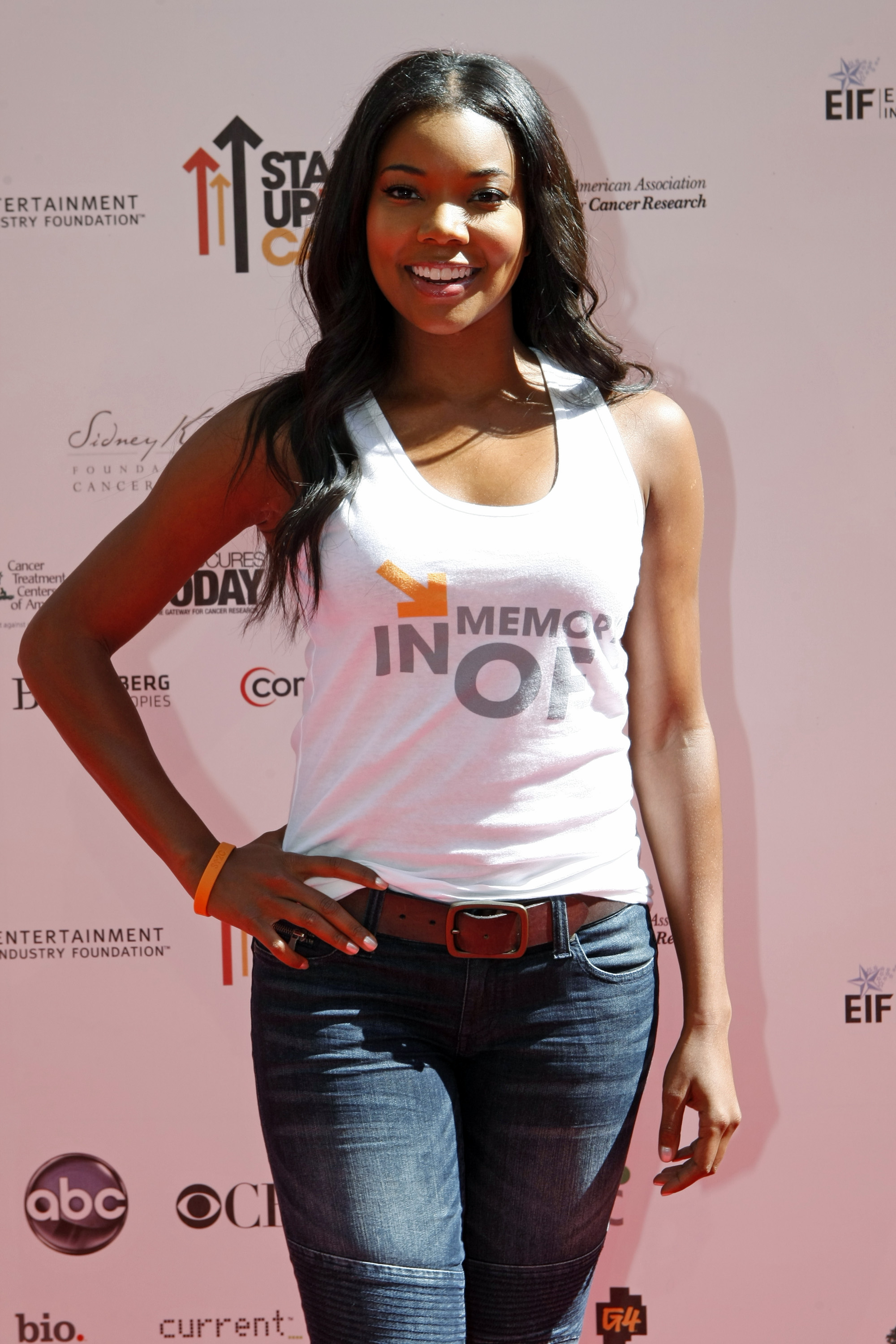The image features a young woman standing in front of a white backdrop adorned with various logos, including those of ABC, CBS, and Comcast. Prominently displayed are logos for the American Association for Cancer Research and Stand Up To Cancer, which features upward-pointing arrows. The backdrop also includes an EIF logo. At the center of the image, the woman, identified as Gabrielle Union, is posing confidently with one hand resting on her hip. She is dressed in a sleeveless white tank top that bears the inscription "In Memory Of," paired with blue jeans and a leather belt. Her long, dark hair cascades below her shoulders, and she is wearing an orange bracelet on the hand at her hip. Gabrielle Union is flashing a broad smile that reveals her teeth, clearly enjoying the moment.